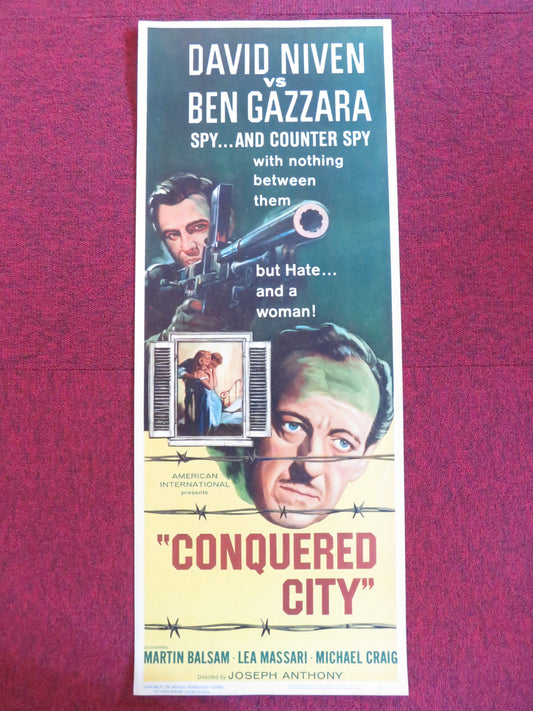The image is a full-color, vertically rectangular movie poster set against a horizontally rectangular, textured purple and blue background. At the top of the poster, bold text reads: "David Niven vs. Ben Gazzara: Spy and counter-spy with nothing between them but hate and a woman." Below this, there is an illustration of a man holding a long rifle, positioned towards the middle top of the poster, with the rifle pointing to the right. Just beneath this scene is a window frame showing a man and a woman in an embrace. Further down, towards the bottom right of the poster, a man's face is prominent with strands of barbed wire crossing over it. The title "Conquered City" is prominently displayed near the bottom, with the names of the actors Martin Balsam, Lea Massari, Michael Craig, and the director Joseph Anthony listed at the very bottom. The poster expertly combines elements of intrigue and romance, encapsulating the dramatic essence of the film.